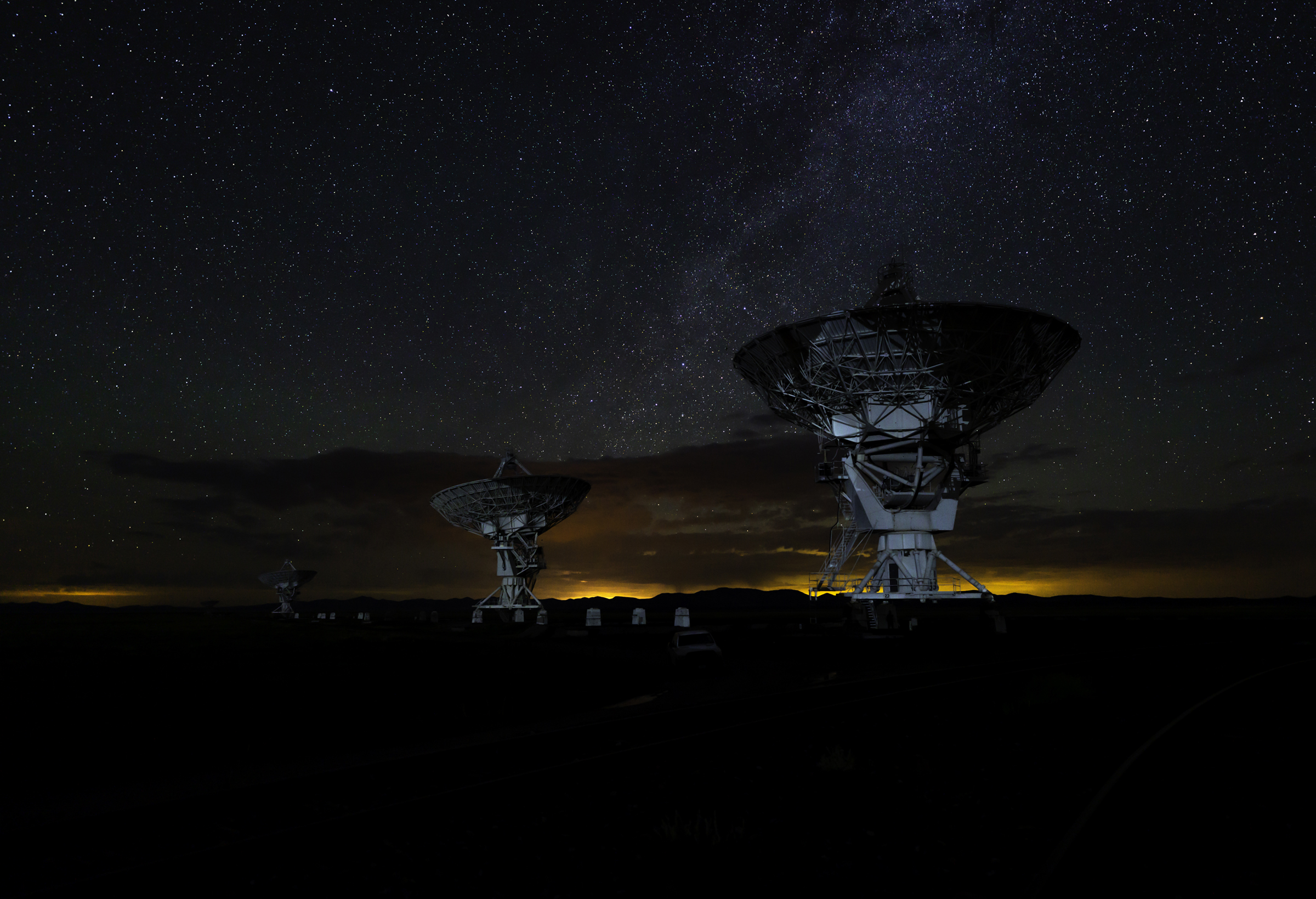The image showcases three large satellite dishes, resembling antennas, positioned on Earth under a night sky. The photo, which could be from a video game, a 3D creation, or real life, features one prominent satellite dish on the right, with two smaller dishes trailing off into the distance on the left. Each dish is constructed from white metal, characterized by intricate steel girders forming a triangular pattern at their centers. All three satellite dishes are directed upwards.

The scene is captured at night, with a pitch-black foreground contrasting against a horizon awash in golden yellow hues, suggesting the sun is either setting or rising. Above, the crystal-clear sky is dotted with thousands of white stars, with light clouds interspersed, adding to the celestial beauty. The overall atmosphere evokes a sense of watching a scene from a science fiction movie like "Contact," blending the mystery of space with the precision of advanced technology.